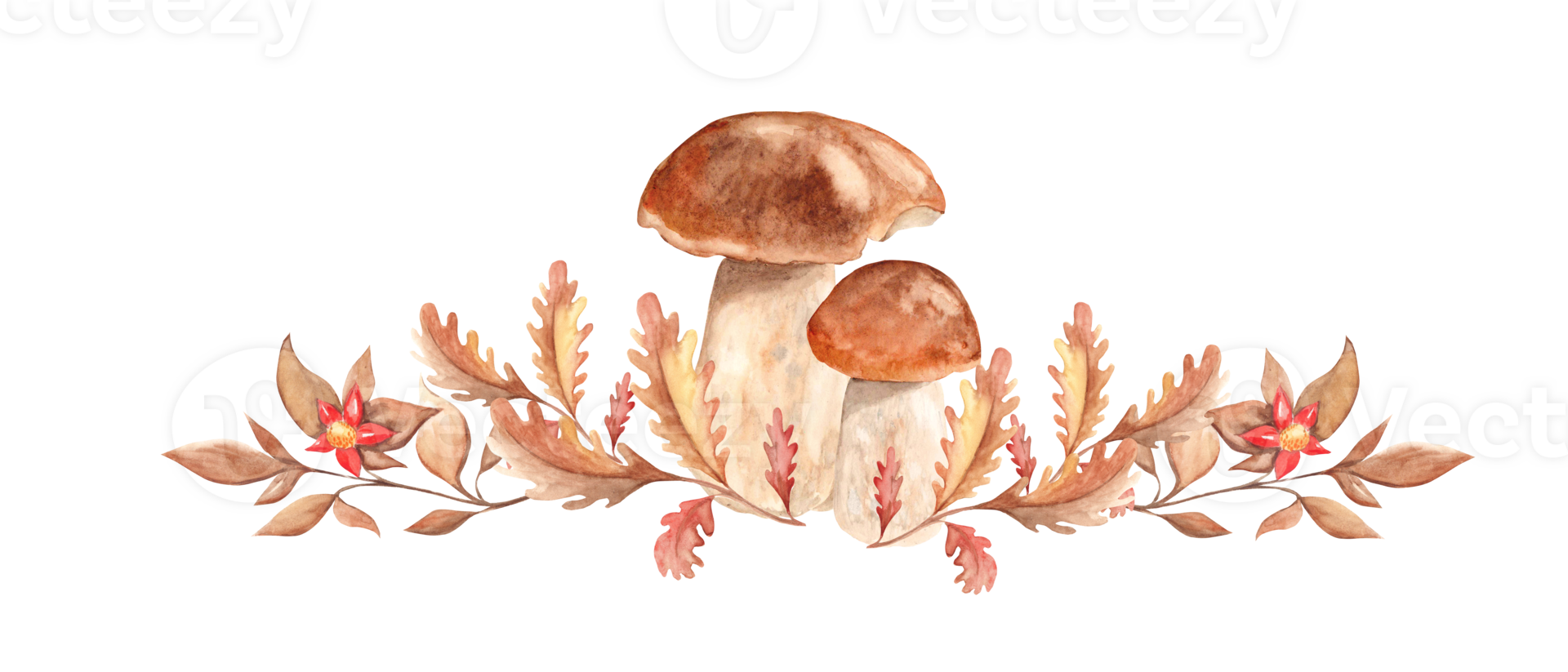The image displays a detailed print on a pure white background, featuring two centrally positioned mushrooms. The mushrooms stand side by side, with the larger mushroom on the left and the smaller on the right. Both mushrooms have thick, off-white stems and sandy, reddish-brown caps. The larger mushroom has small imperfections on its cap, including a bite-like mark. Surrounding the base of the mushrooms are clustered oak leaves and other pointy-edged leaves in autumnal hues of orange, brown, tan, and rusty reds. Symmetrically placed near the leaves are red and yellow flowers, adding a vivid contrast. The entire scene appears as if the mushrooms and foliage are suspended in midair, and faint portions of text are visible near the top of the image. The artwork's dimensions suggest it is notably wider than it is tall, enhancing its landscape orientation.